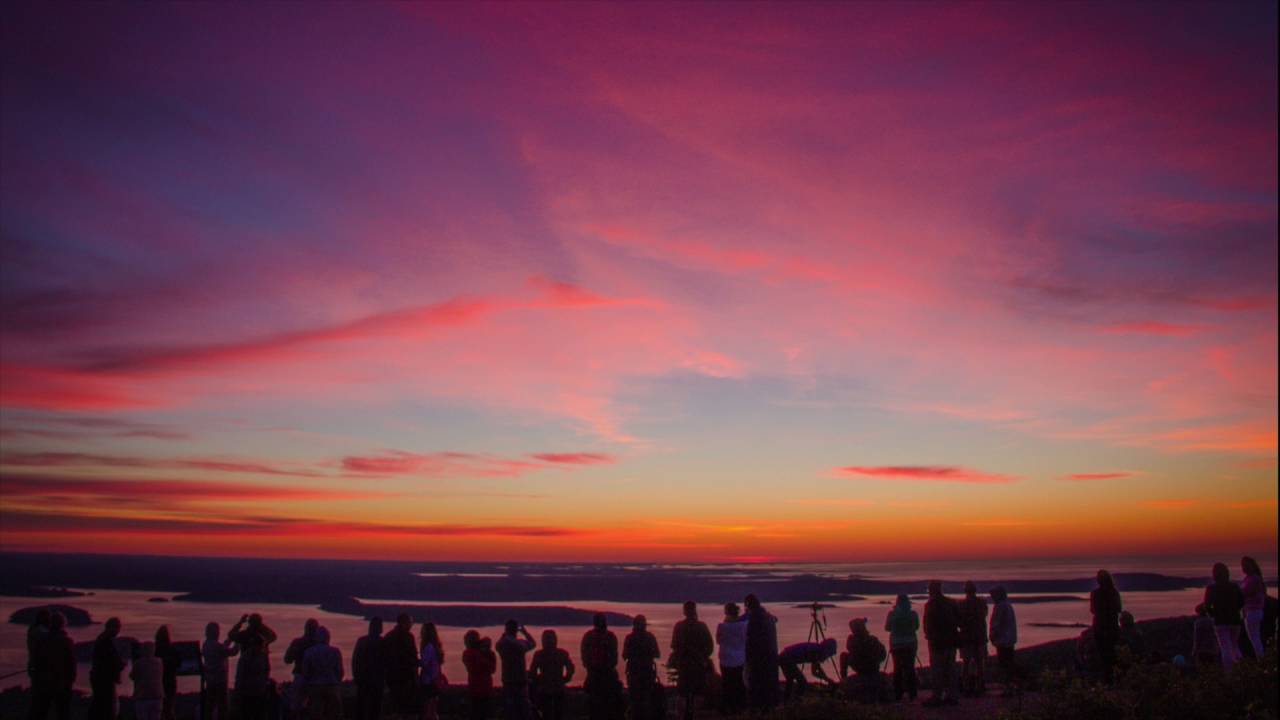In this captivating photograph taken during either sunrise or sunset, a large group of over a dozen people stands in silhouette, their backs facing the camera, gazing across a tranquil body of water towards the sky. The sky dominates the frame, painted with a breathtaking array of colors—deep red, vibrant orange, soft pink, and hints of blue—highlighting the ethereal beauty of the moment. The water below them reflects the fading or emerging light, adding a serene mirror-like quality to the scene. Islands and a distant coastline are faintly visible, adding depth to the composition. The clouds, illuminated by the sun’s rays, further enhance the scene with their pink and orange hues. The overall effect is a stunning depiction of nature's grandeur and the peaceful coexistence of these silent observers with the natural spectacle unfolding before them.